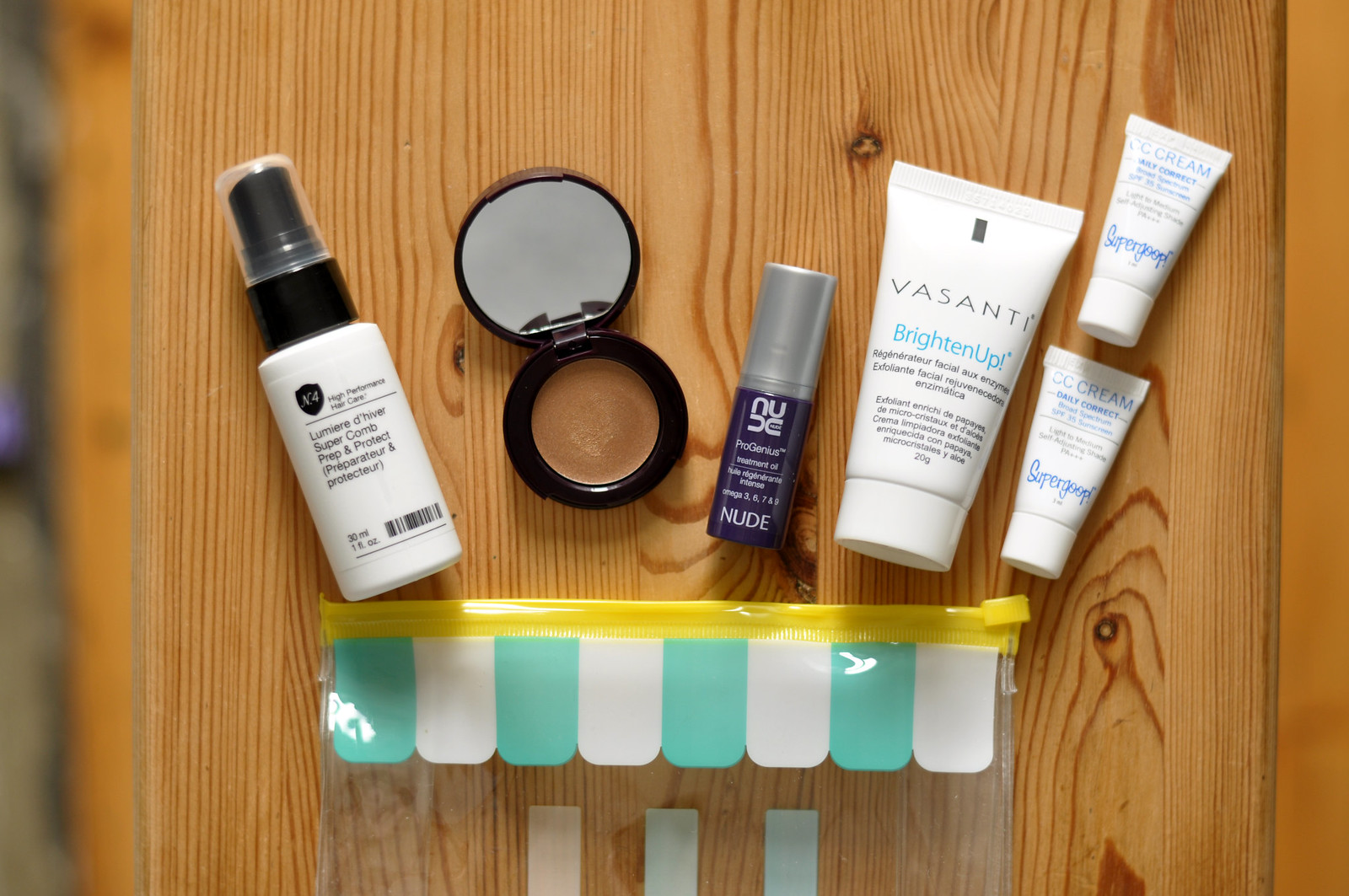The image portrays a clear travel bag with teal and white stripes, featuring a yellow Ziploc seal, placed on a wooden table. The bag contains essential personal care items and some makeup products, likely intended for a vacation. Arranged from left to right, there is a spray bottle of hair product, an unidentified makeup item, a nude-shaded product, a facial moisturizer, and two containers of Supergoop sunscreen. Most items are housed in white bottles with screw-on caps. Additionally, there is a blurry object on the far left edge of the table. The items are neatly centered and aligned towards the bag in a top-down perspective.